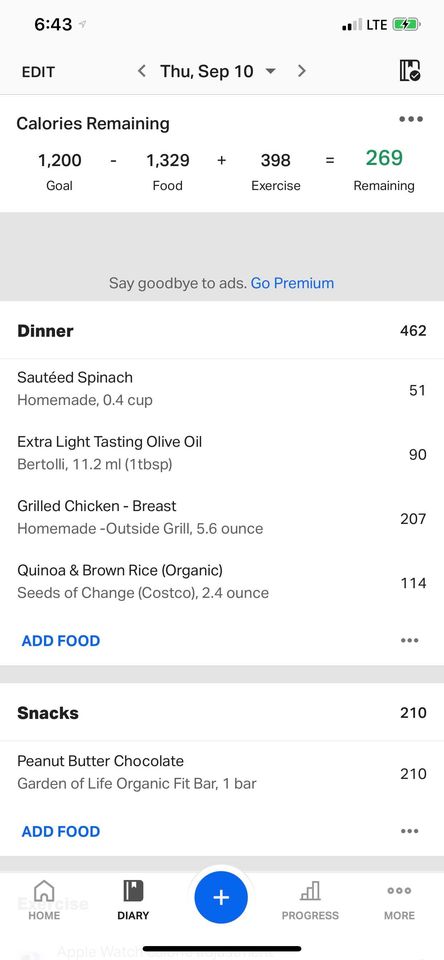The image depicts a mobile application screen likely designed for diet tracking or recipe management. The interface indicates today’s date as Thursday, September 10th.

At the top, there is a calorie summary:
- **Calories Remaining:** 269
- **Calories Goal:** 1200
- **Calories Consumed:** 1329 (Food)
- **Calories Burned:** 398 (Exercise)

Below the summary, there is a prompt offering an upgrade to a premium version to remove ads.

Further down, the app details dinner intake:
- **Dinner Total:** 462 calories
  - **Sautéed Spinach:** 51 calories 
    - *0.4 cups homemade sautéed spinach*
    - *1 tablespoon (11.2 ml) Bertoli extra light tasting olive oil – 90 calories*
  - **Grilled Chicken Breast:** 207 calories 
    - *5.6 ounces homemade, grilled outside*
  - **Quinoa and Brown Rice:** 114 calories 
    - *2.4 ounces, organic Seeds of Change from Costco*

Snacks are also logged:
- **Snack Total:** 210 calories 
  - *1 Garden of Life organic fit bar, peanut butter and chocolate – 210 calories*

At the bottom of the screen, there are navigation buttons labeled "Progress," "More Info," "Diary," and "Home," allowing users to access different sections of the app.